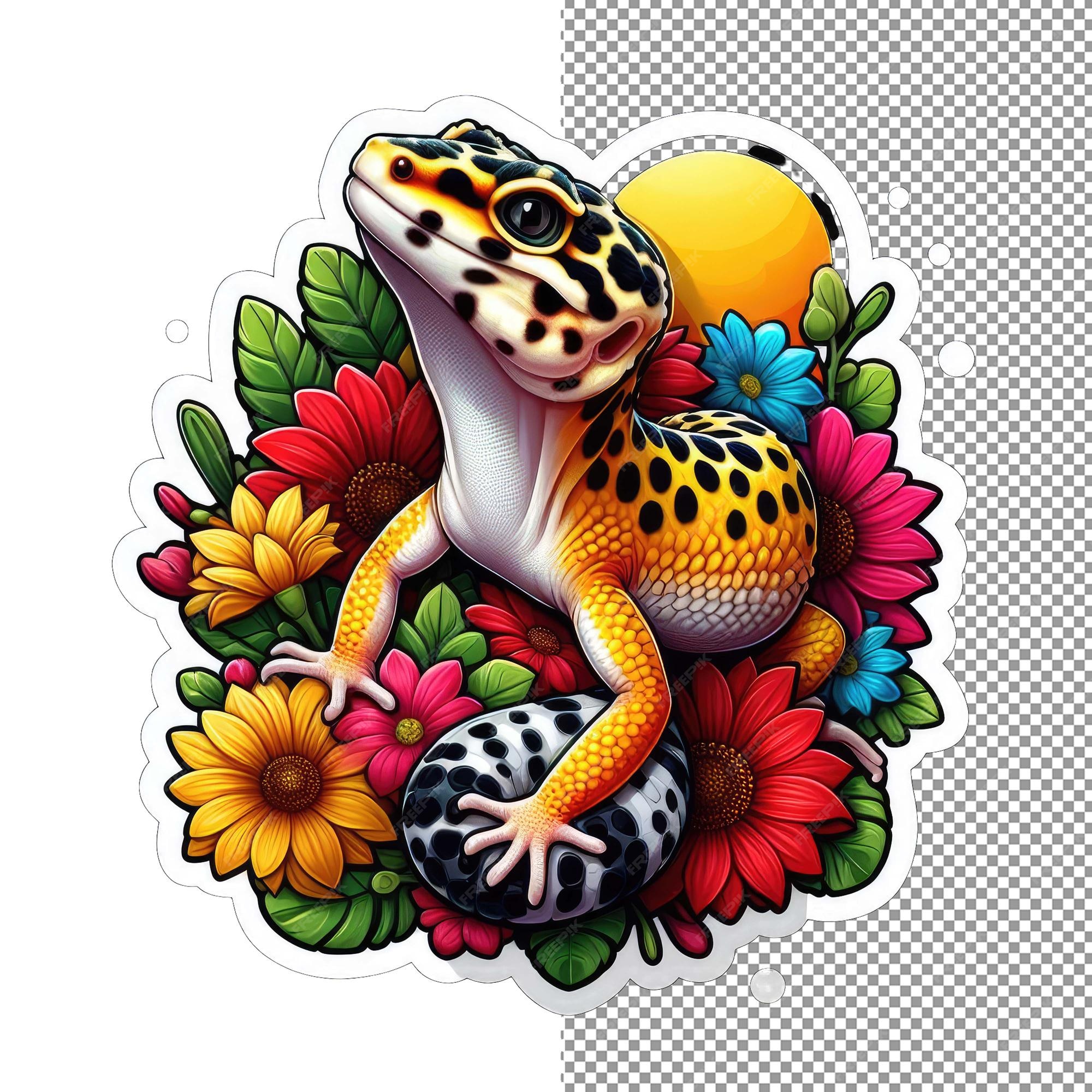The image features a vibrant digital print of a gecko at the center, appearing as a colorful sticker. The gecko has a white belly, with its back and legs adorned in yellow scales speckled with black dots. It is depicted climbing over various flowers and leaves, with its head tilted towards the top left. The flowers surrounding the gecko are in hues of red, yellow, pink, blue, and magenta, while the leaves are a bright green. Under one of its paws lies a white stone with black dots. Behind the gecko, there is a yellow circular shape resembling the sun. The background is divided: the left half is plain white, while the right half features a gray and white checkered pattern, emphasizing the image's digital nature. The gecko’s body is positioned to the right with its arms extended in front, encapsulated by the floral and leafy sticker design.